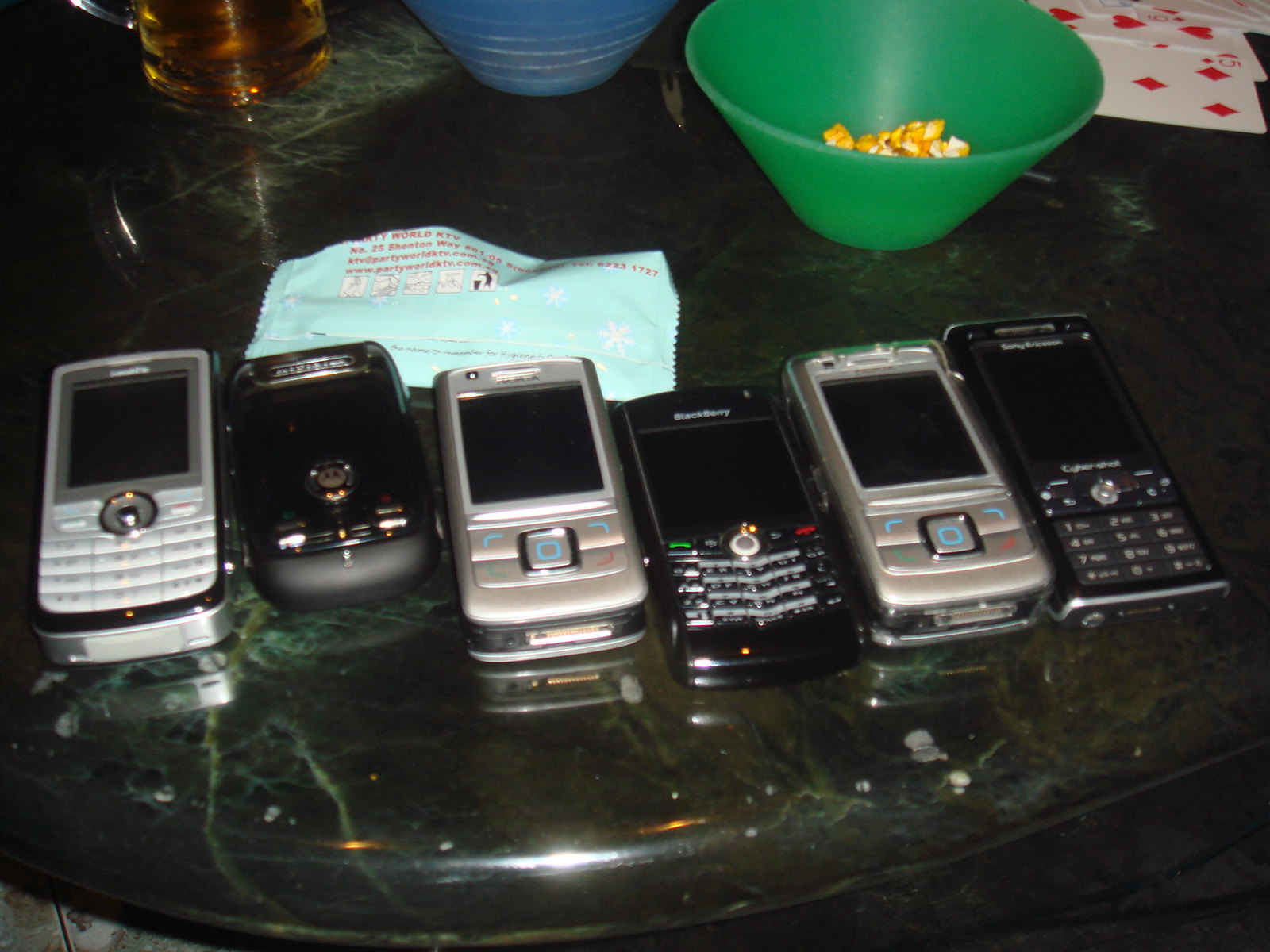This photograph showcases a collection of six early-generation mobile devices arranged on a dark, circular granite table with a greenish hue. From left to right, the devices include a thick bar-style phone in silver with a white face and a large central button, a black Motorola flip phone with silver accents, a silver sliding phone with minimal buttons resembling a Blackberry, another thick silver phone with just four buttons and one central button, a black phone with a standard keypad featuring a green and red button on either side, and another silver phone similar to the third one. The background reveals a casual setting with a bag of candy, a drink cup, the lower half of a clear bottle with a warm amber-brown liquid, a blue ridged bowl, a green plastic bowl containing a small amount of cheddar-flavored popcorn, and a few scattered playing cards on the table. None of the phones' screens are turned on, highlighting their dormant, nostalgic state.